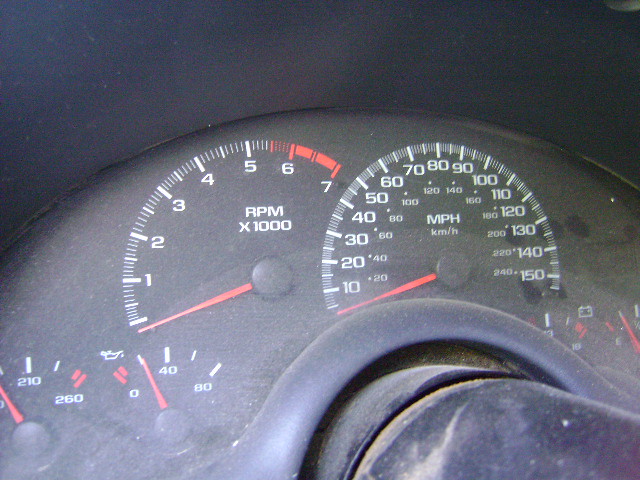This image showcases the dashboard of a vehicle, featuring four prominent gauges with intricate details.

1. **RPM Meter (Rev Counter)**: This gauge is positioned prominently, with its scale ranging from 0 to 7, marked off in single increments. The sector between 5.5 and 7 is highlighted in red, warning of high RPMs. The meter's pointers are a vivid red, and the hash marks for every RPM are described, with thicker markings at each whole number.

2. **Speedometer**: Encircling the right side of the dashboard, it displays speeds from 0 to 150 mph in 10 mph increments, although the '0' is not labeled. Inside the mph scale, kilometers per hour indicators are marked in a smaller font. All numerical values and hash marks are in white against a black background, with the pointer also colored red.

3. **Oil Pressure Gauge**: Located next to the speedometer, this semicircular gauge presents readings at 0, 40, and 80 (presumably in psi), also featuring white numerals on a black background, with the needle in red. 

4. **Unknown Gauge**: On the bottom left of the image, this gauge is partially visible and displays the number '210' at the center and '260' at the far right, with the leftmost portion cut off. The details are somewhat unclear, but it follows similar design conventions with white numerals and a red pointer.

Each gauge maintains a uniform aesthetic with black backgrounds and white text, except for the red zoned warning areas on the RPM meter. The dials’ pointers are consistently red, making them easily readable against the black and white backdrop.